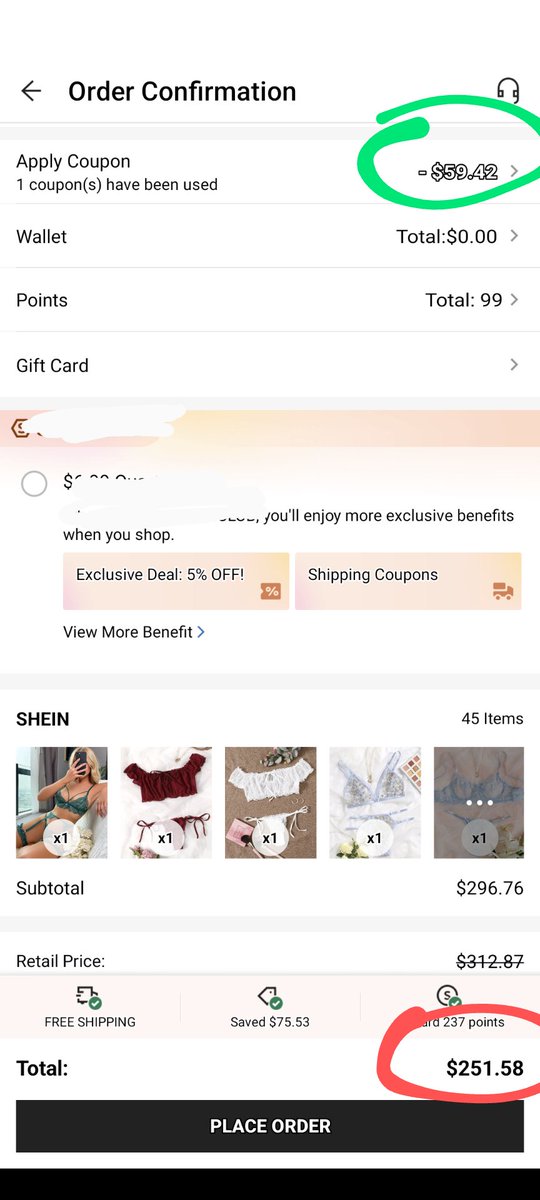The image depicts an order confirmation screen with a clean, white background at the top. Centered and in bold black text, it reads "Order Confirmation." In the top left corner, there is a left-pointing arrow icon. 

Below this section, a gray strip spans the width of the image, after which the background returns to white. The text “Apply Coupon” appears in black, and beneath it, smaller text notes "1 coupon(s) have been used."

On the right side of this section, prominently displayed in large, blocky numbers, is the amount "$59.42," encased in a black outline and circled with a green marker. 

A faint gray line divider follows, under which the word "Wallet" appears in bold black text. To the right, it states "Total: $0.00," with an arrow pointing to the right. Another divider line is below this.

Next, the section labeled "Points" appears, and to the right, it states "Total: 99." This is followed by another divider, under which "Gift Card" is listed, with an arrow on the right suggesting further navigation.

The bottom part of the screen is headed by a section with an ombre color gradient, transitioning from peach to yellow in the middle. The top text of this section is scratched out with white. Below, a bubble is outlined in light gray with a price inside, whited out as well. Under this, in small black text, reads the phrase, "When you shop."